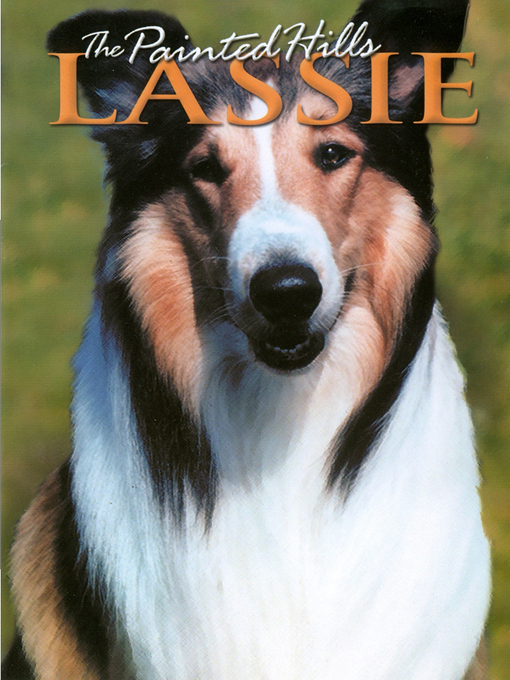The magazine cover features a close-up image of a large shepherd breed dog, centered against an outdoor daytime backdrop, indicative of being taken in a field of grass. The dog, presumably sitting on its hindquarters, showcases a distinct tricolor coat: primarily brown with patches of black and white fur. Its face is light brown, accented by a white spot around its nose and mouth, and both its dark eyes are looking forward. The dog’s pointed ears add to its attentive gaze, though its left ear is slightly drooping. Text is overlaid on the photograph, with "The Painted Hills" written in a small, white cursive font nestled between the L and the I of the much larger and bolder, orange 3D-styled word "Lassie." The colors present in the photo, including blacks, whites, browns, and touches of green from the grass, make for a vibrant yet clean composition suitable for a family-oriented magazine cover.